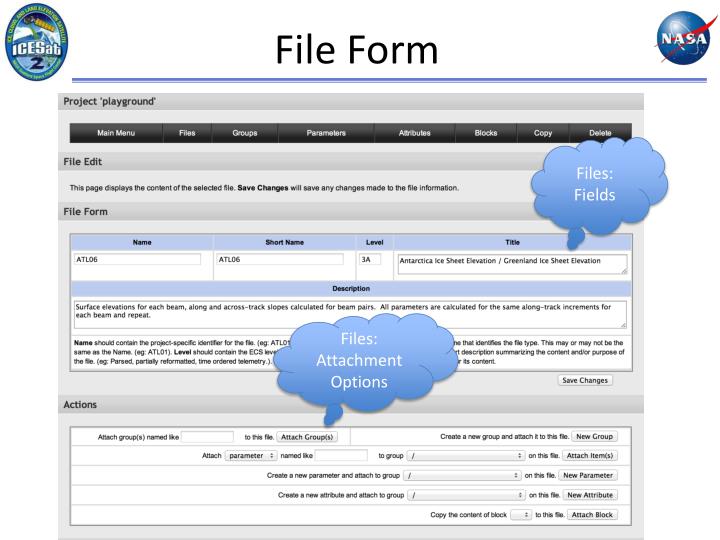The image depicts a detailed application form displayed on a computer screen, likely a phone, laptop, or desktop. At the top left is an insignia labeled "ICESat," featuring an egg shape with a mountainous background. In the top right corner is a circle displaying the NASA logo. Centered between these logos, the title "File Form" is prominently displayed with a blue underline. Beneath the title is the project name "Project Playground."

The interface is predominantly gray with blue accents, and a menu bar runs across the top containing options such as Main Menu, Files, Groups, Parameters, Attributes, Blocks, Copy, and Delete. The form itself includes fields for key information like Name, Short Name, Level, and Title, all highlighted with blue. Two blue clouds provide additional guidance: one pointing out "Files Fields" and the other "Files Attach Options." At the bottom of the form, under a section labeled "Actions," there are more spaces available for additional inputs. The structured layout suggests the form is utilized for detailed data entry, possibly in a NASA-related project.